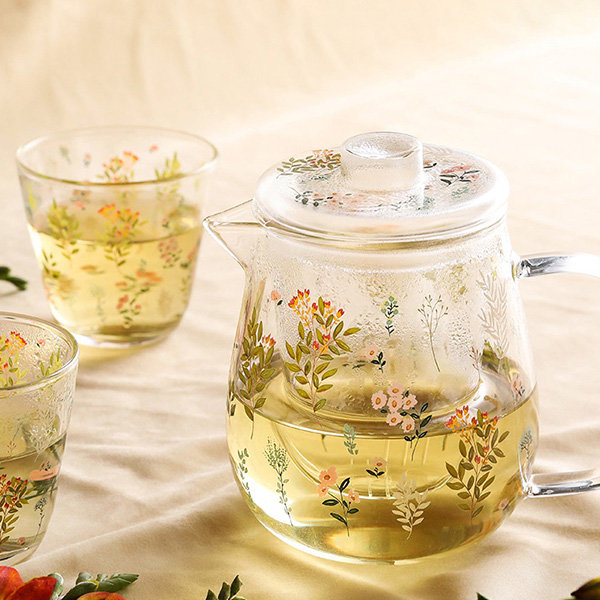The image showcases a beautifully arranged tea set. A prominent, clear glass teapot with a handle and lid is filled halfway with a delicate, light yellow tea. The teapot features intricately hand-painted floral designs, with pink flowers, green leaves, some white flowers with yellow petals, and smaller orange flowers interwoven in the pattern. The serene floral motif continues onto two clear glass teacups without handles situated near the teapot. Both cups are also half-filled with the same light yellow tea, and the cup on the top left appears to be 70% full. The set is elegantly placed on a white tablecloth that drapes from the floor up onto the wall, creating a soft beige-tan backdrop. Adding a touch of natural beauty, scattered red flower petals and green leaves decorate the bottom left corner of the scene.